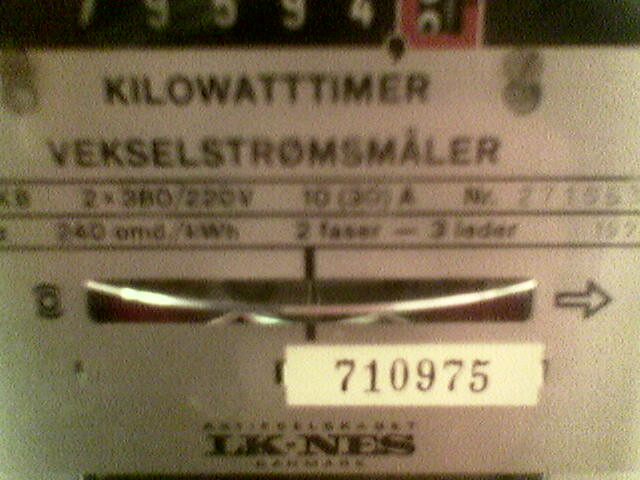This image is a zoomed-in, somewhat blurry photograph of an electricity meter, used to measure kilowatt usage, likely taken with a phone. At the top of the meter, the label "Kilowatt Timer" is prominently displayed, indicating its function. Below this, there is a long word in a foreign language, "VEKSELSTROMSMALER," suggesting technical specifications. Underneath, detailed information about voltage appears: "2 x 280/220 volts, 10 (30) A." The meter has a rotating dial displaying the current kilowatt reading. Notably, a silver plate on the meter features a white sticker with the number "710975." At the bottom of the meter, there is a logo reading "LKNES," with "Denmark" noted next to it, all text rendered in black font against a white background. This device resembles those typically attached to homes for monitoring by power companies.